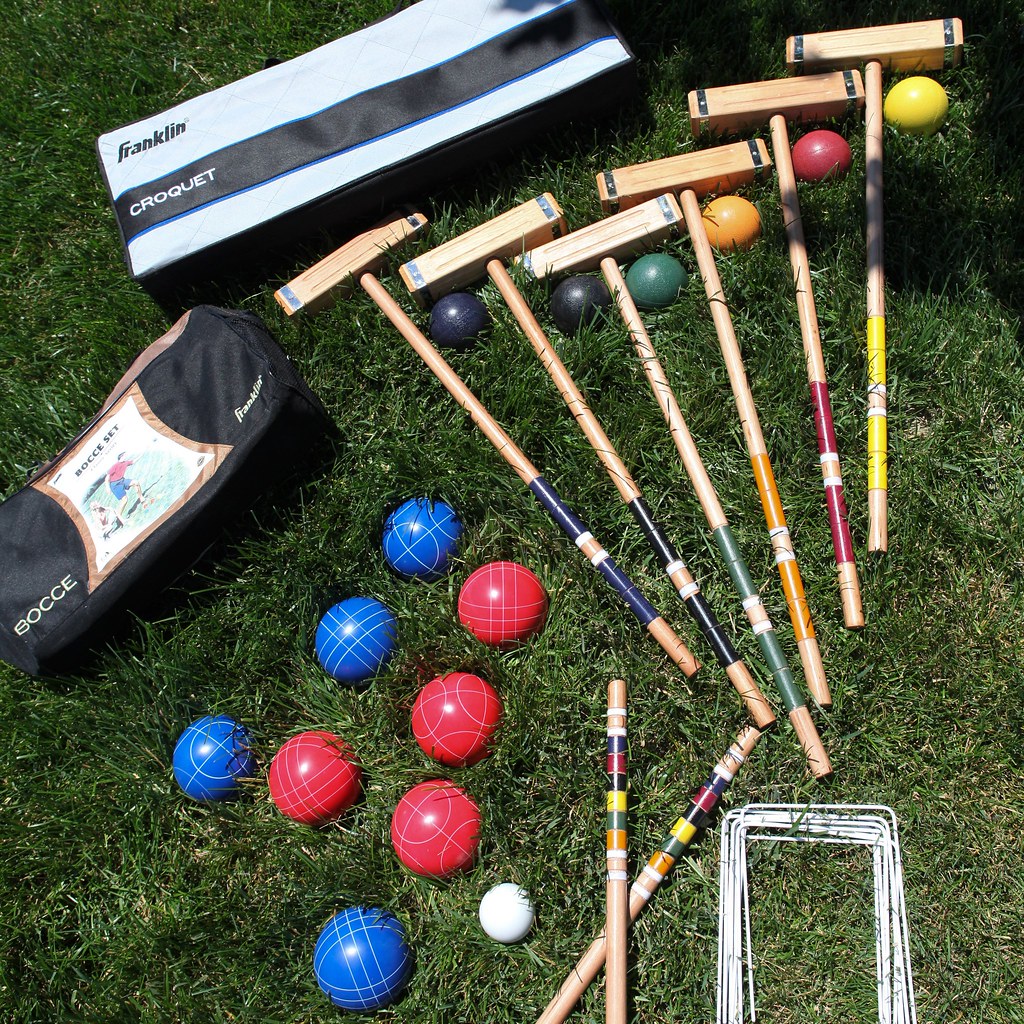This image depicts a vibrant croquet and bocce set laid out on a grassy area with mild patches of brown in the bottom right corner. At the top, six croquet mallets are organized in a neat row, each separated by a different colored ball—yellow, red, orange, green, black, and dark blue. In the bottom left corner, eight croquet balls are arranged, evenly split between red and blue. Among them is a small white ball, part of the bocce set. Two croquet sticks are crossed at the bottom, near white metal goal posts (wickets) intended to be staked into the grass. In the top left corner, there are two rectangular bags: the upper one is blue and black striped with “Franklin Croquet” branding, while the lower black bag, labeled “Franklin Bocce,” features an emblem of a man playing bocce. The detailed arrangement and variety of colors and equipment underscore the dual nature of the game sets ready for play on this lush, albeit slightly patchy, grass field.